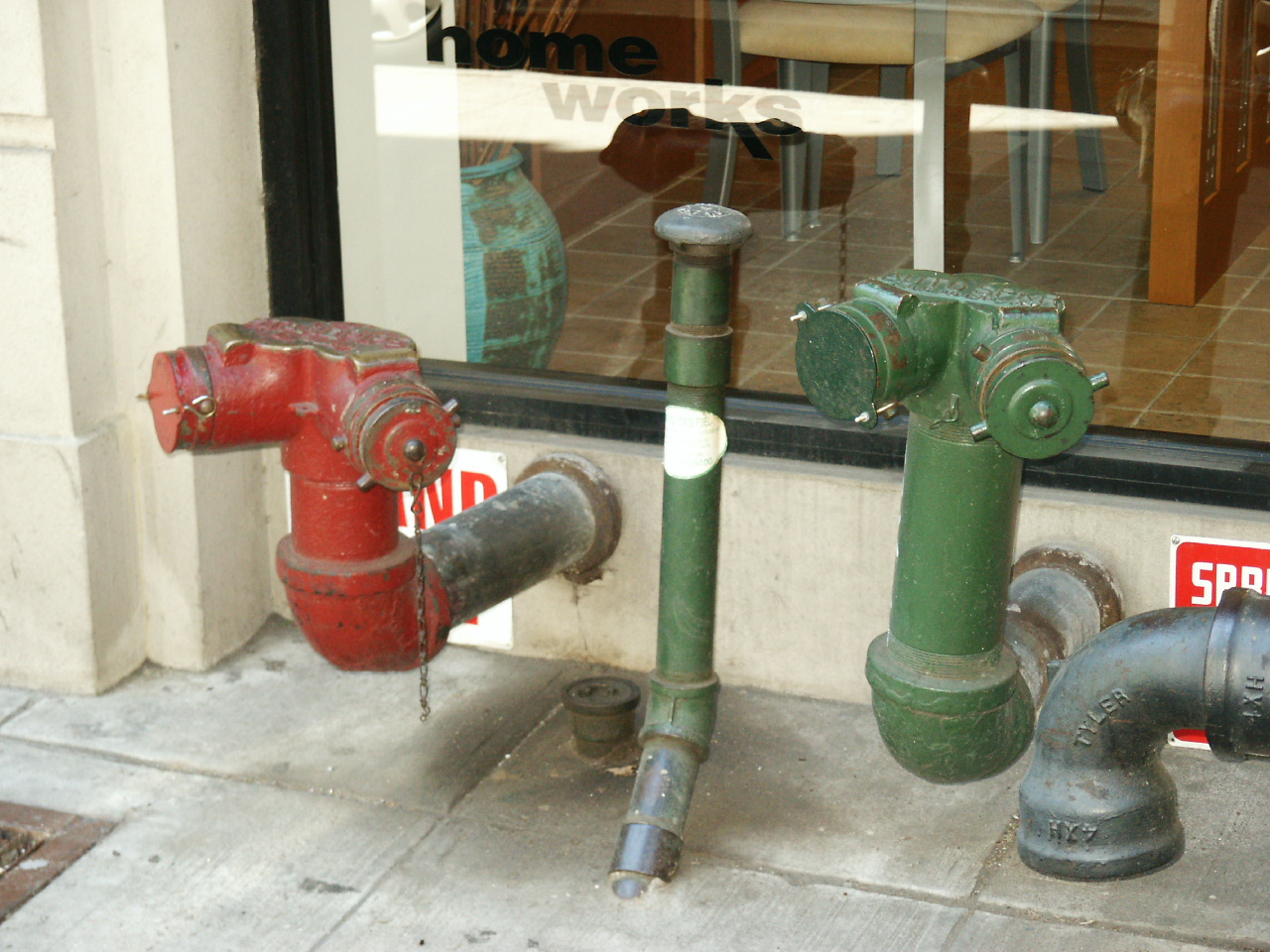This vibrant color photograph captures a bustling city sidewalk scene on a sunny day. The grey concrete sidewalk is lined with prominent metal pipes, predominantly painted red, green, and black. Two L-shaped fire hose connections project from the side of a cement-colored building: the left one is red with twin spigots, while the right, taller one, is green with similar dual spigots. At the center of this street-side display, a taller green standpipe emerges directly from the sidewalk. Completing the quartet of urban plumbing, a substantial elbow-shaped black pipe points downward from the lower right-hand corner of the scene. Above these intriguing utility fixtures, a window reflects the city's activity and offers a glimpse inside the building, revealing a chair and an ornate urn-like vase. The word "WORKS" is clearly visible on a white rectangular piece of acetate affixed to the window, adding a layer of character and context to the urban landscape.